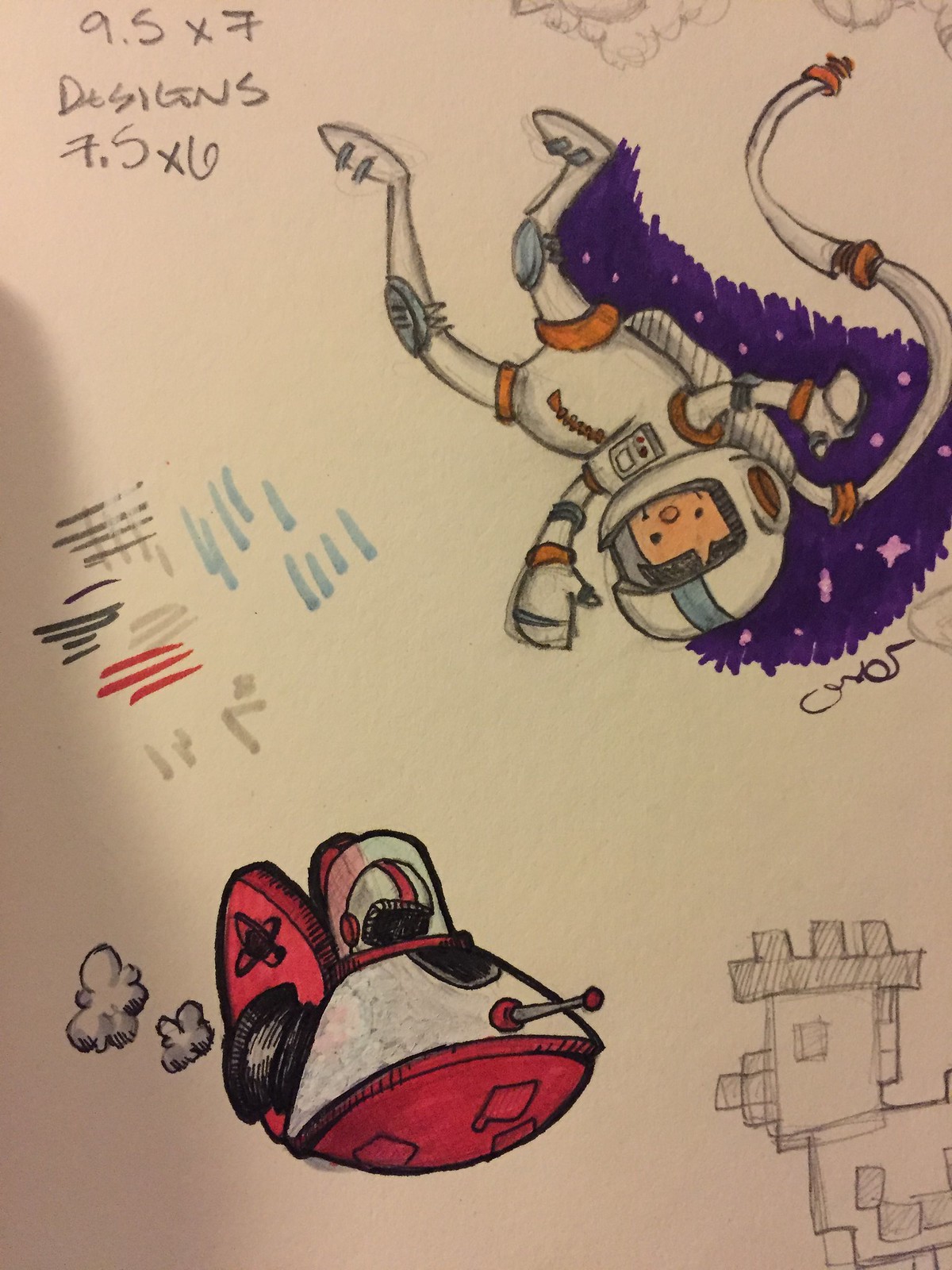The vertical drawing presented is a detailed sketch and layout of an illustration, likely intended for a cartoon. This professional-grade artwork features several figures meticulously rendered on paper. 

At the top, penciled-in dimensions read "9.5 by 7." Central to the image is a cartoon spaceship reminiscent of the iconic Jetsons' design, completed with intricate pen and ink work. The spaceship is adorned with red and gray shading and emits two puffs of smoke from its rear. A person's helmet can be seen inside the craft, adding a touch of character.

In the upper right corner, there is an upside-down astronaut tethered to something off-frame. The astronaut, who bears a striking resemblance to Calvin from the comic strip Calvin and Hobbes, is intricately outlined in pencil. Surrounding him is a vibrant scene featuring orange, blue, and purple hues, set against a backdrop dotted with light purple stars.

In the bottom right corner, a robot dog is sketched in pencil, partially entering the frame. The sketch also includes some marker lines, suggesting preliminary color planning or additional detail work. The combination of pen, ink, pencil, and marker lines, along with the professional quality of the drawing, creates a visually engaging and complex illustration.